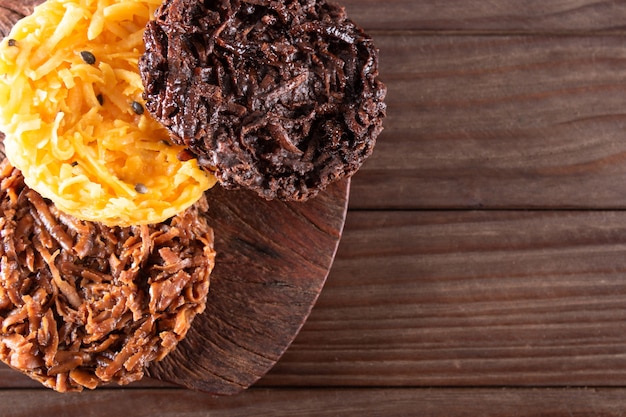The photo showcases an overhead view of a rich, dark wooden table with a round wooden plate placed off to the left side. On the plate, there are three distinct and separate circular food items, each with a unique texture and color. The item at the bottom appears to be meaty, while the one in the middle has a cheese-like appearance with a yellow hue, possibly indicative of a vanilla or butterscotch flavor. The top right item is dark brown, likely a chocolate or coconut caramel cookie. These items are thin, suggesting a crispy texture. The backdrop comprises rectangular wooden panels, adding a natural, earthy tone to the setting, with no additional text or indicators of the environment or time of day.